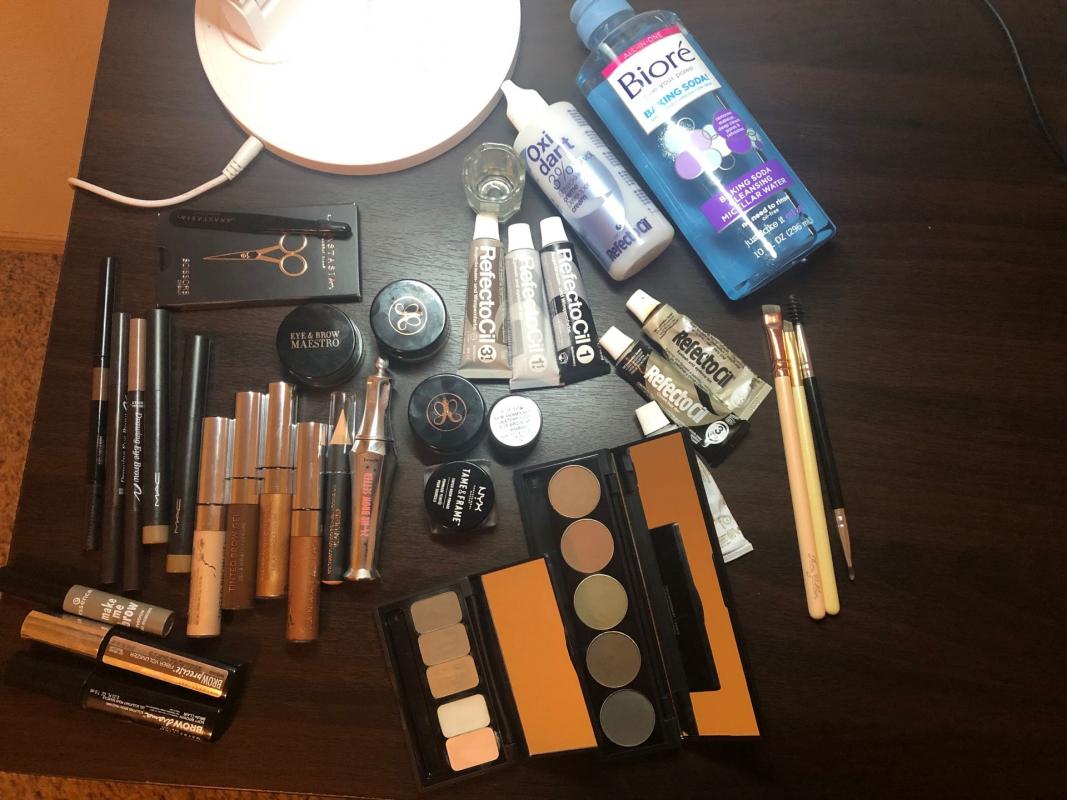A meticulously arranged collection of makeup and facial products is displayed on a dark brown table. The scene is illuminated by a bright light, the base of which is partially visible, casting a well-lit glow over the array. On the right side of the table, several makeup brushes are neatly laid out. Nearby, a pair of tweezers and a pair of scissors are placed, ready for precise grooming. Among the assorted cosmetics, a selection of closed lipsticks and mascaras awaits use. Prominent in the scene are a few specific products: a bottle labeled 'Oxydart' with a visible '3%' mark, a 'Biore Baking Soda Cleansing Water,' and a 'Refecto Oil.' Additionally, two different black makeup palettes—one containing circular pans and the other, rectangular—are open, revealing an array of shades in gold, brown, beige, and various skin tones. The detailed organization suggests a professional or enthusiast's workspace, ready for makeup application or experimentation.